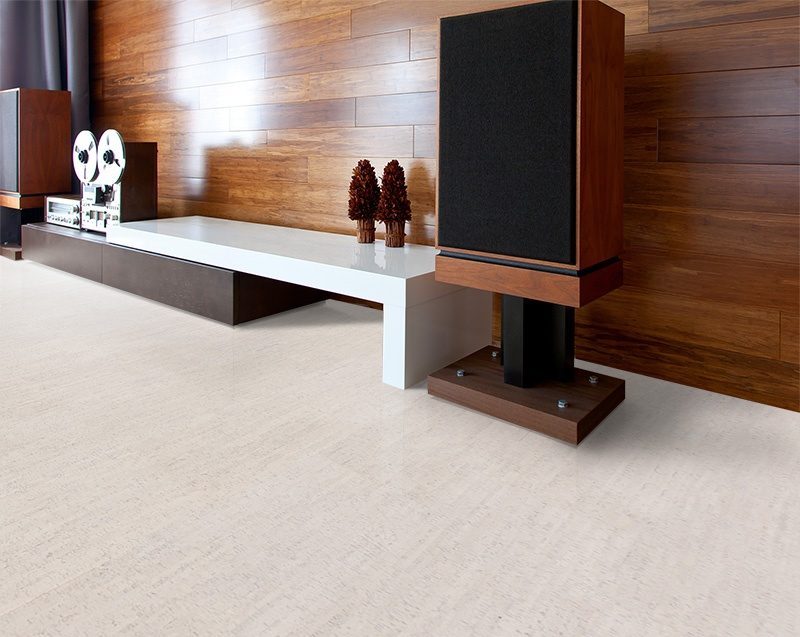The image depicts a room with a dark brown wooden wall adorned with light reflecting off of it. Against this wall is a long white table or TV stand, which lacks a television set. Flanking the table are two large wooden speakers with black audio fronts, resting on a light beige or off-white floor. To the left of the composition hangs a rippled, dark red curtain. Adjacent to the speakers is an old sound machine, possibly a vintage radio player, which sits beside the white table. The scene is detailed with additional elements like circular details on the speakers, silver nuts on the speaker stands, and a brown object resembling a flower vase atop the table.